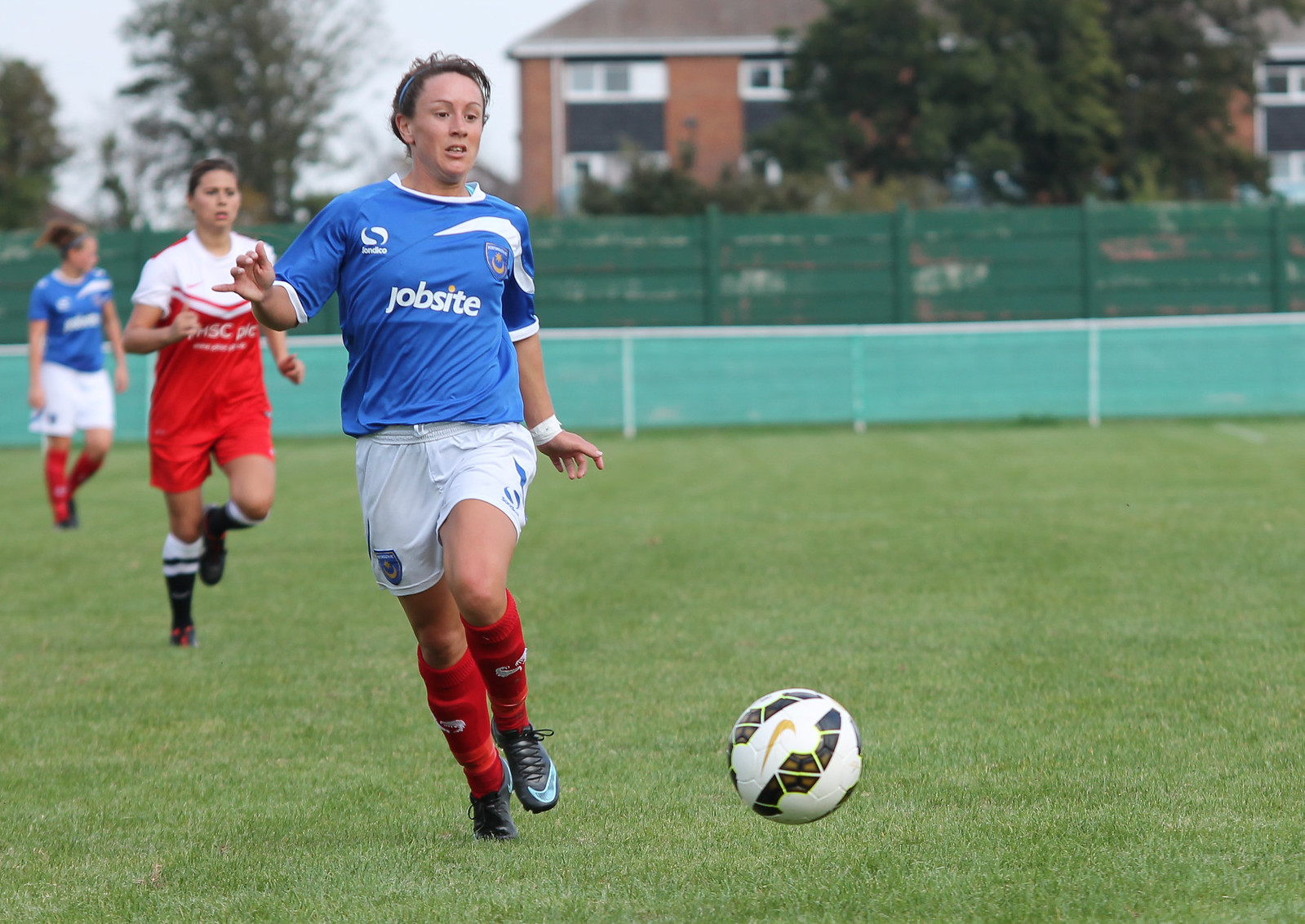The horizontal rectangular photograph captures an action-packed scene in a soccer match featuring female players. Three players dominate the left side of the image, two in blue shirts and white shorts with red socks and black shoes, and one in a red and white top, red shorts, and black socks. The foremost blue player is sprinting toward a white soccer ball adorned with a Nike checkmark logo and darker stripes, centered in the lower middle part of the photograph. 

The background showcases a green playing field without visible yard markers, suggesting an indefinite position on the pitch. Behind the players, a green fence—with a lighter green bottom and a darker green top—frames the scene. Beyond the fence, dense trees partially obscure a tall brick building with numerous windows framed in white, hinting at it being residential or possibly an office building. The overall composition combines dynamic athletic movement with a subtly detailed and slightly blurred backdrop, focusing on the intensity of the match.